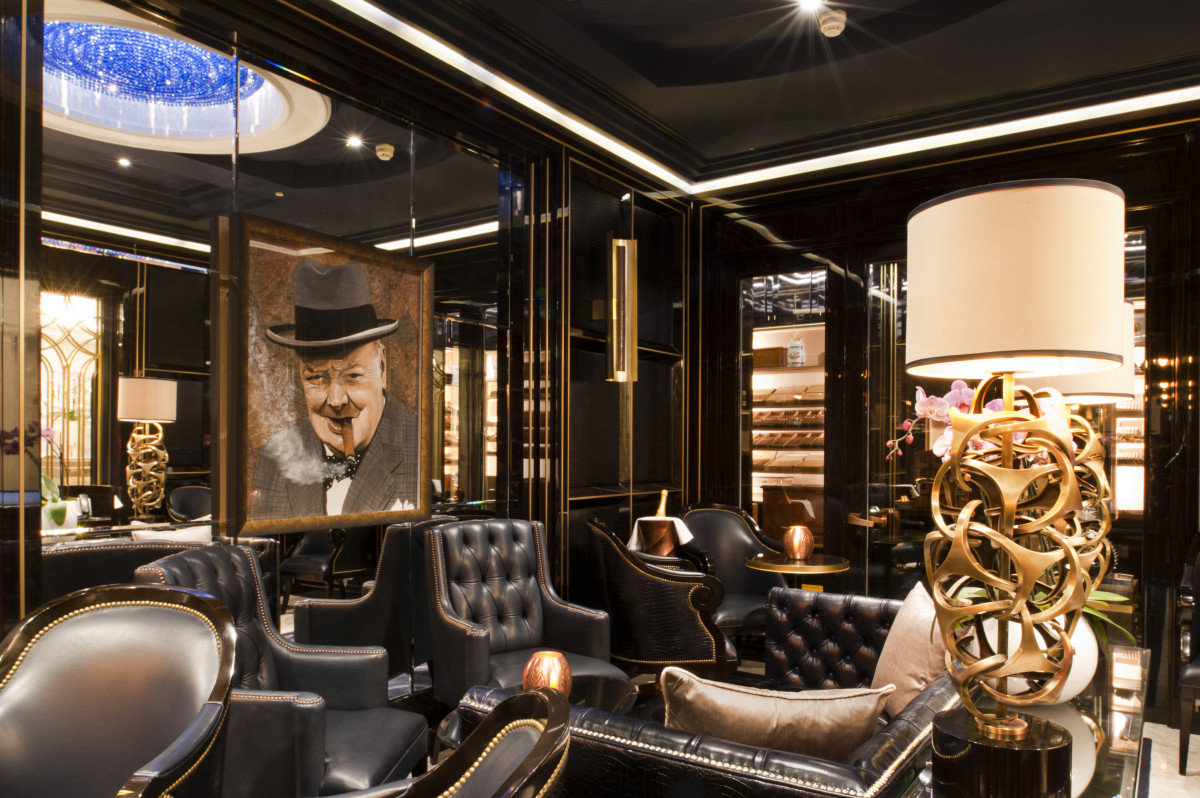The image depicts the interior of a luxurious lounge, evocative of an old-fashioned smoking club. The room features numerous black leather armchairs and carefully detailed decor. On the left, a striking black and gold-trimmed wall hosts a picture of a man who resembles Winston Churchill, complete with a gray plaid suit jacket, a top hat, and a lit cigar with smoke curling upwards. Adjacent to this image, the shiny surface could either be a mirror or a window reflecting parts of the room. The chairs throughout the room have gray cushions, black wood borders, and gold bead trim that adds to the room's opulence. On the right side of the image, there's an ornate lamp on an oval table, its base crafted from interconnected gold pieces, resembling antlers, with a white lampshade casting a warm yellow glow. The room is cloaked in a dark, rich ambiance, amplified by the shiny black ceiling with a perimeter light, giving the impression of an upscale, empty men’s club.